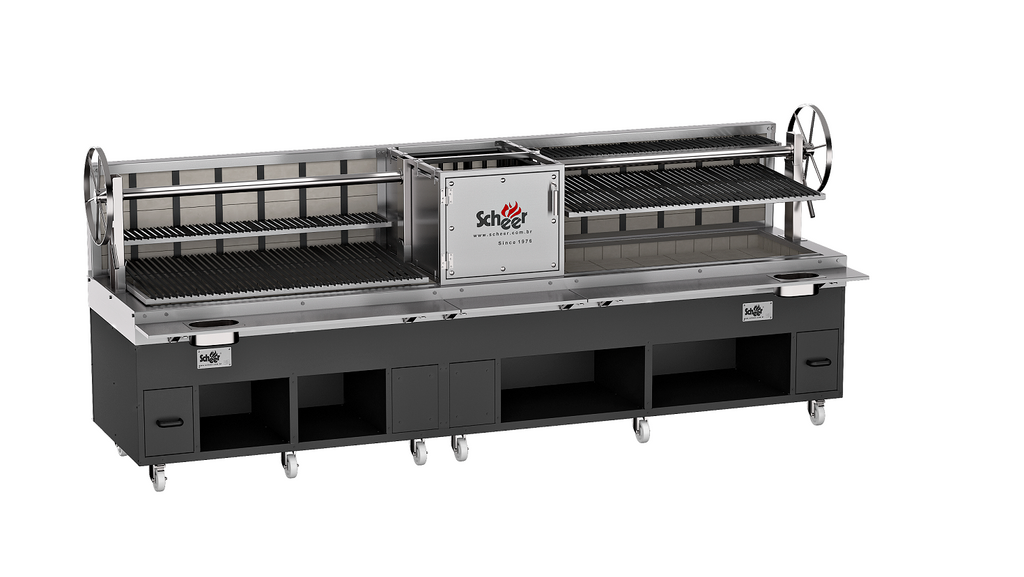This is a detailed product photo of a large industrial grill by Scheer, S-C-H-E-E-R, set against a clean white background. The massive stainless steel equipment features a functional design with a black base and white wheels for mobility. Central to its operation are two large metal wheels on either side, which allow the adjustable grill grate to be raised or lowered closer to or further from the fire. The grill is built for heavy-duty cooking, possibly in a commercial or fast food restaurant. 

Beneath the grill sits ample shelving and storage, encased in the black cabinet, all built atop a set of wheels for easy movement. Adding to its versatility, the grill includes a flat-top on the right side for different cooking techniques. Above the primary grill section is an additional grill grate, suggesting it could support rotisserie functions, ideal for cooking items like burgers, hot dogs, or rotisserie chickens. 

The overall length of the grill is approximately 10 feet and about 3 feet deep, making it a substantial addition to any industrial kitchen. The branding is prominently displayed with "Scheer" and a flame logo, emphasizing its cooking-related purpose, along with a website address and a note of establishment since 1976, indicating a long history in the industrial kitchen equipment market.

Additionally, the design includes practical elements such as trash disposals with designated holes in the countertop area for quick waste disposal, along with a functional silver backsplash to maintain cleanliness and safety. This versatile and sizeable piece of equipment is undoubtedly built for professional culinary environments, offering flexibility and efficiency for various cooking needs.